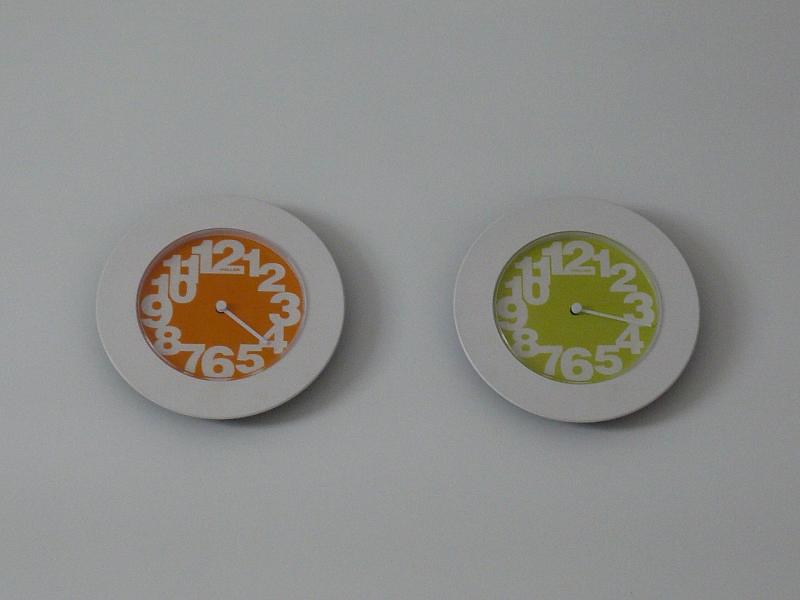This photograph captures a dimly lit wall with a grayish hue. The wall is adorned with two circular clocks that blend into the wall due to their similarly colored gray rims. The clock on the left features an orange face with white numbers and hands, indicating the time as four o'clock. The clock on the right, set some distance apart from the first, showcases a lime green face, also with white numbers and hands, displaying the time as approximately three-thirty. The minimalistic image focuses solely on these two distinctively colored clocks, standing out against the otherwise plain background.